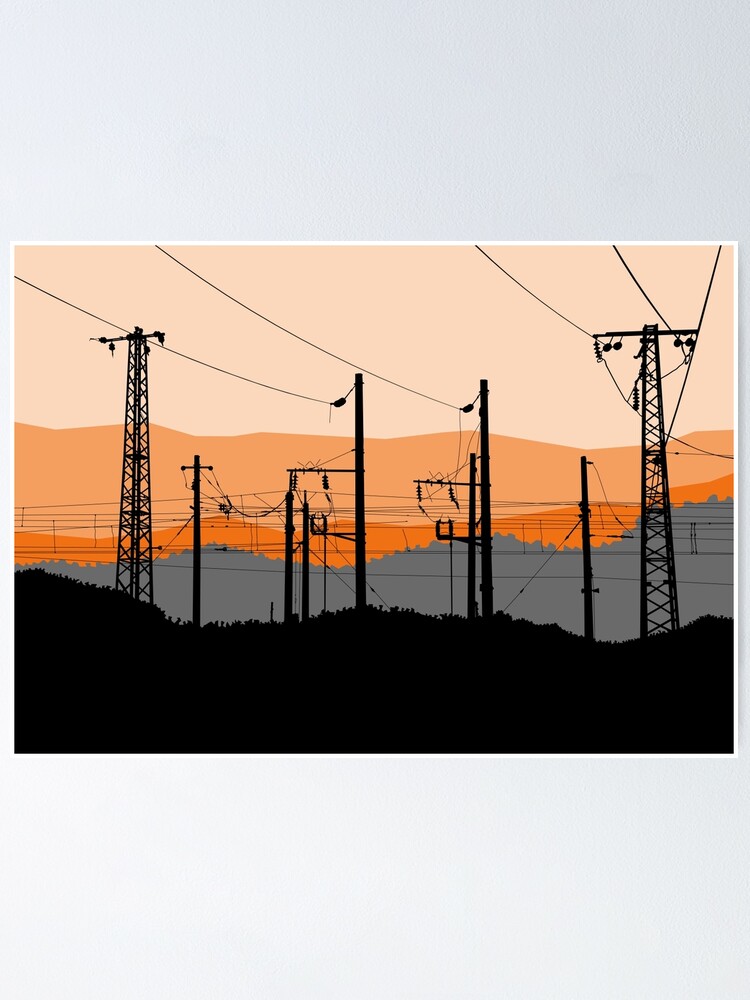The image appears to be a highly detailed print or painting, mounted against a gray background with a narrow white border. The main focus of the picture is the high transmission power lines in the foreground, silhouetted in black. These lines undulate across the image from left to right, some supported by steel uprights with insulators and cross arms, while others are held by tall wooden posts. The wires themselves crisscross the scene, adding a dynamic, somewhat chaotic element. 

In the lower portion of the image, silhouettes of grass or low bushes can be seen. Behind the power lines, there's a progressively lighter gradient of colors: starting with a dark gray band resembling hills that grow taller as they move from left to right, followed by a thin layer of dark orange, which indicates either a sunset or distant mountains. Above this, a larger expanse of a lighter orange suggests a range of mountains or foothills, transitioning into a very pale orange sky, almost a light pink salmon hue, indicative of a setting sun. The entire scene, artistic and industrial in nature, is suggestive of a sunset over a landscape dotted with power lines and hills, depicted mainly through silhouettes.